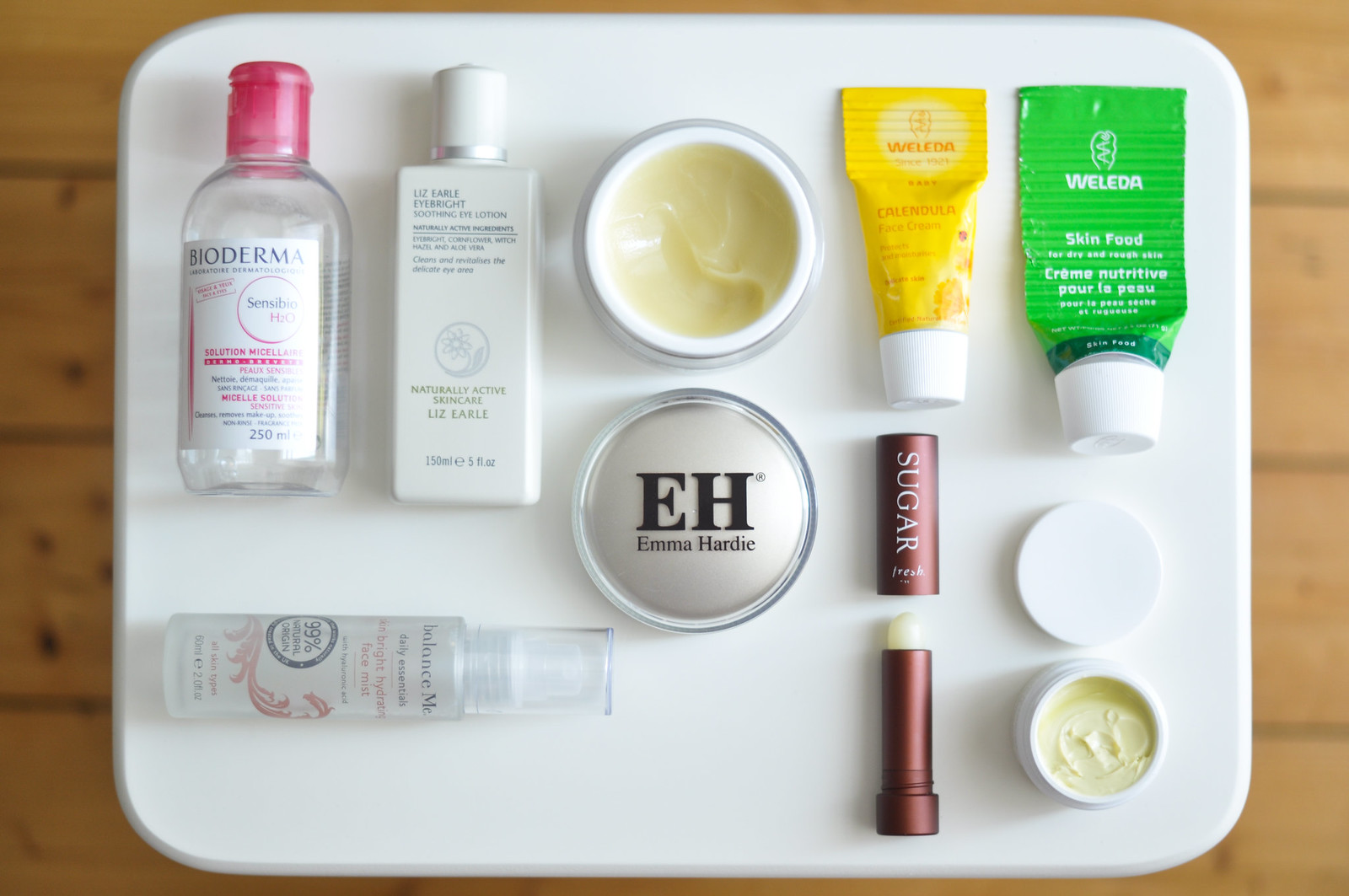A diverse collection of skincare and makeup products is artfully arranged on what appears to be a wooden table, with a white wooden cutting board or palette featuring rounded corners as the backdrop. In the upper left corner, there is a clear bottle with a red top labeled "Bioderma." The label is somewhat blurry, making it difficult to decipher the smaller text. To its right, a tall, vertically rectangular bottle marked "naturally active skincare" from Liz Earle, with a white cap, is noticeable. This bottle contains 150 milliliters of product. 

Below these, there's a white tube, although the brand or product name isn't visible. Adjacent to this, there is a circular container labeled "Emma Hardy" with the initials "E.H." Next to it, a yellow bottle from Weleda is positioned, followed by a green bottle from the same brand, identified as "Skin Food."

In the bottom left corner, a clear bottle is placed, but its contents are not easily readable. To its right stands a burgundy tube which appears to be a lipstick labeled "Sugar." Finally, another container of cream is spotted to the far right, with its white lid resting directly above it. The meticulously placed items showcase a rich variety of beauty and skincare essentials.